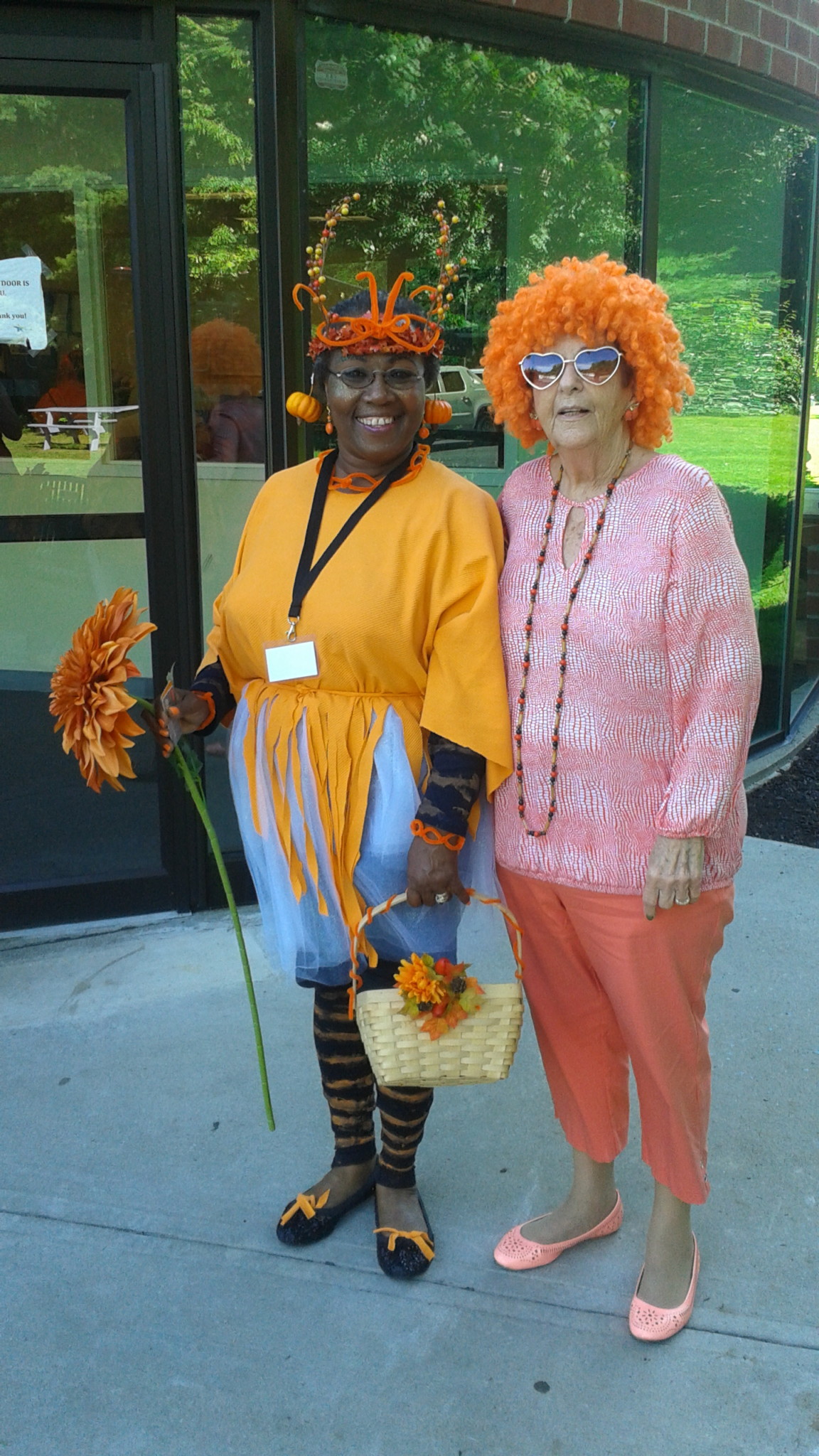This image captures two women at what appears to be a costume event, each adorned in vibrant and playful attire. The woman on the left, who appears to be of African descent, is dressed in an eye-catching ensemble. She wears an orange top paired with a short, bluish tulle dress, complemented by black leggings featuring orange stripes. Her footwear consists of orange and black flats, adding a coordinated touch. She accessorizes with a basket in hand and a decorative headpiece. 

Standing beside her is another woman sporting a whimsical outfit. She is clad in a pink sweater and coral-colored pants, matched with pink flats. Her costume is elevated with an orange curly wig and a pair of heart-shaped sunglasses, completing her fun and festive look. Together, they exude a lively and cheerful vibe, perfectly suited for a costumed celebration.